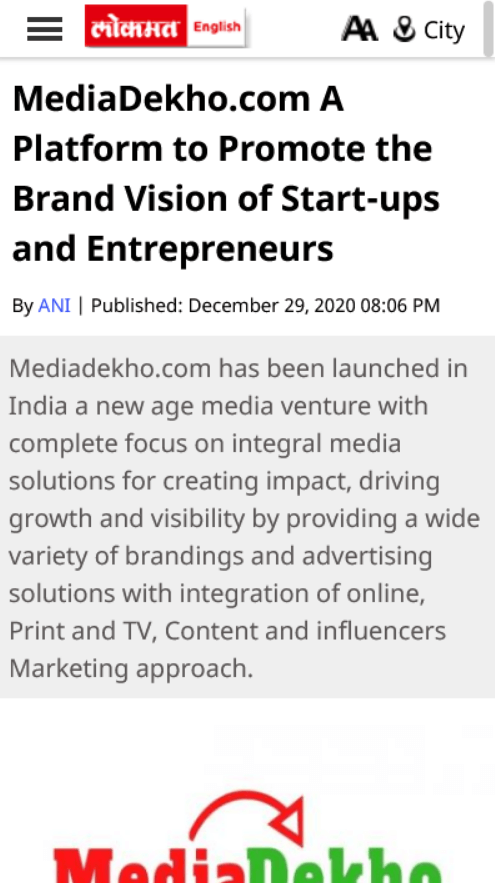**Caption:**

The image is an excerpt from a magazine or newspaper article. It prominently displays information about "Mediadelco.com," a new age media venture launched in India, designed to enhance the brand vision of startups and entrepreneurs. This platform aims to create significant impact, drive growth, and increase visibility by offering a comprehensive suite of branding and advertising solutions. These solutions include integration across online platforms, print, and TV content, alongside influencer marketing strategies. The article was published on December 29th, 2020, at 8:06 PM, and attributed to an author named Annie (styled as "ANI" in blue). Visual elements include the text "AA," a pin indicating a city, and the website "mediadelco.com." The logo at the bottom features "Media" in red and "Delco" in green, connected by a curved red line ending in an arrow pointing from "Media" to "Delco." The header and a section with three horizontal lines in red are also part of the design.